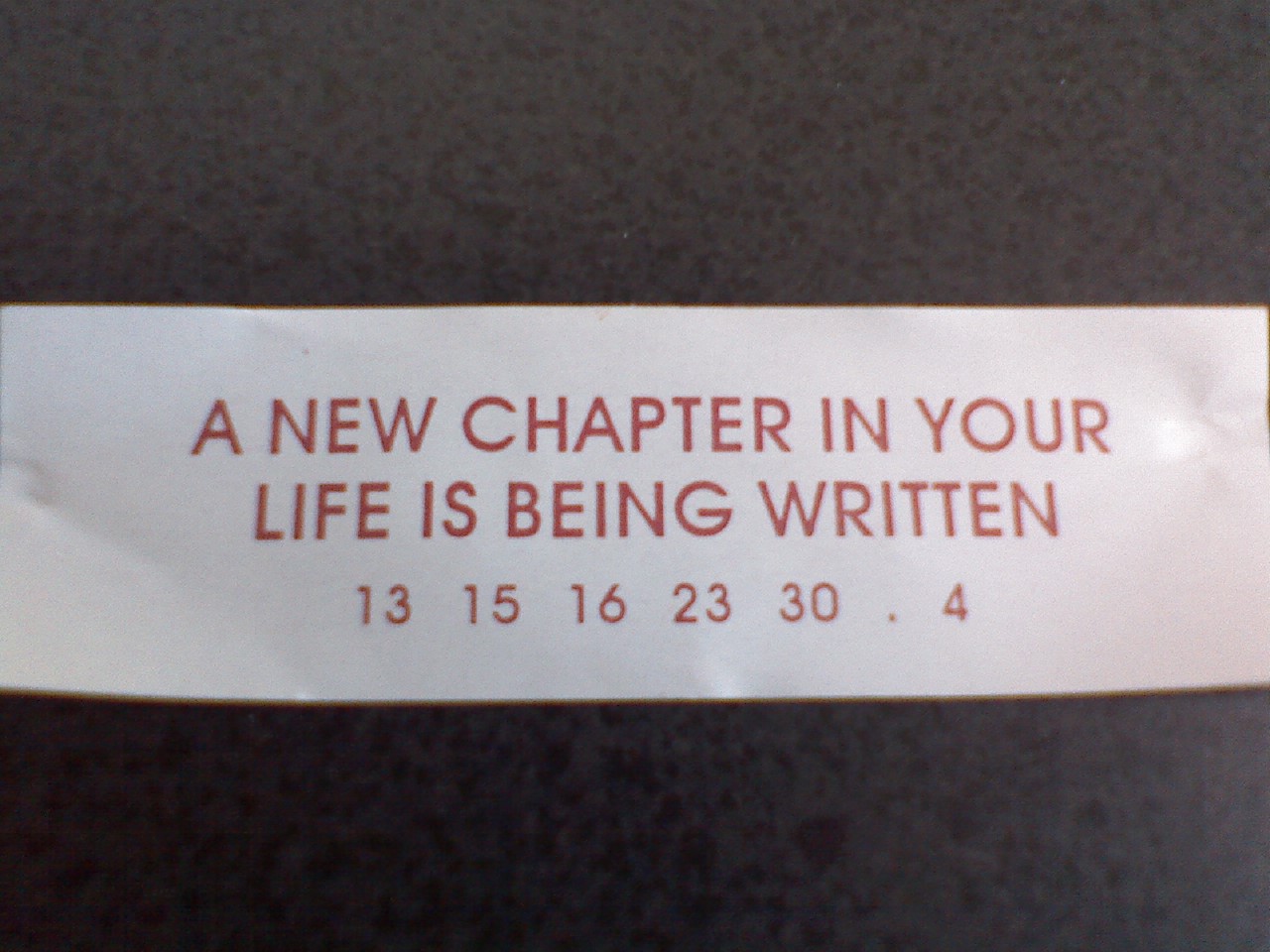The image presents a close-up photograph of a fortune from a fortune cookie, placed against a dark, possibly black or gray, background with subtle smudges and dots. The fortune itself is a narrow white rectangle centrally positioned in the image, extending horizontally from edge to edge. Written in all capitalized red letters, the fortune reads: "A NEW CHAPTER IN YOUR LIFE IS BEING WRITTEN." Below this message, also in red text, is a series of lucky numbers: 13, 15, 16, 23, 30, followed by a period, and then the number 4, suggesting that there might be a missing number.